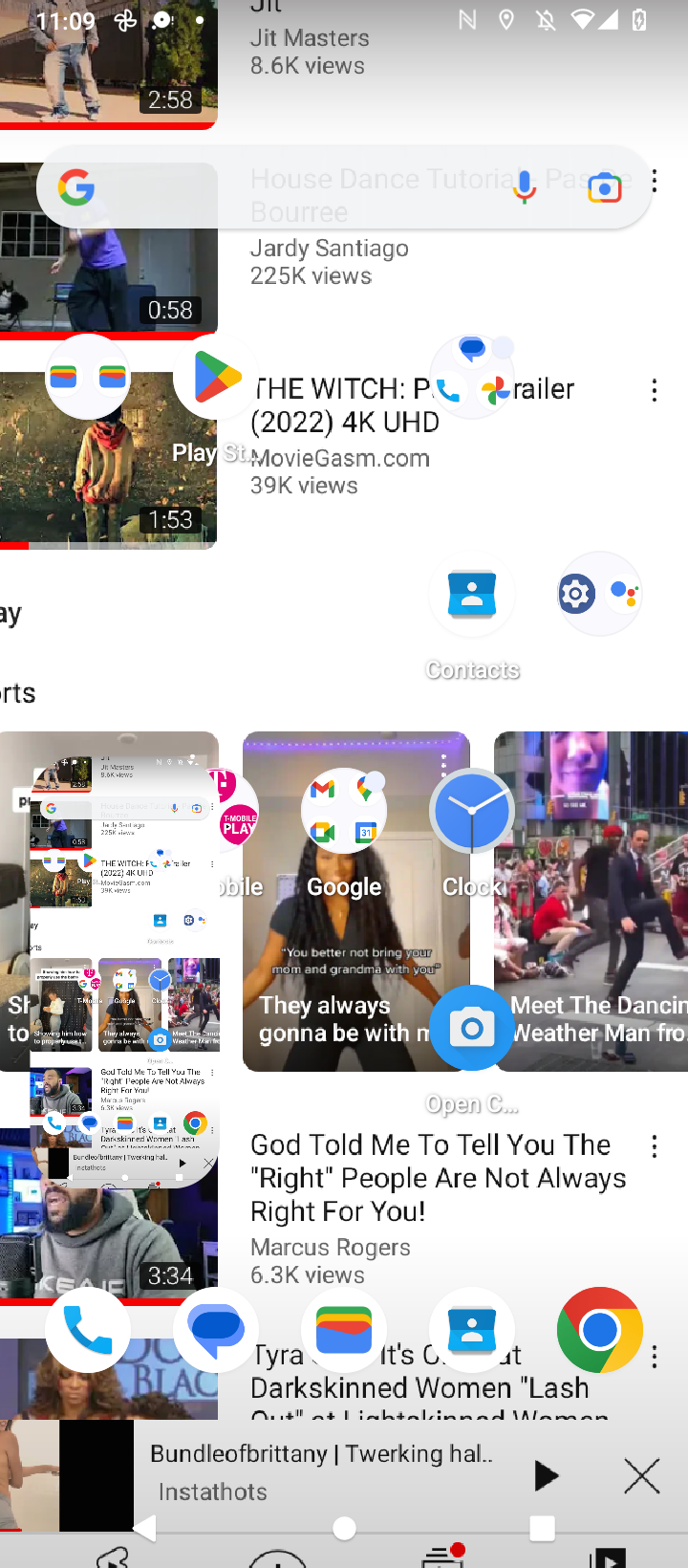The image is a screenshot from a mobile app interface displaying a variety of multimedia content. At the top, there are thumbnails of three videos, each showing the video's title, the creator's name, and the number of views. In one of these thumbnails, the video title reads, "God told me to tell you the, quote, right people are not always right for you," created by Marcus Rogers with 6.3k views. Overlaying this section is a Google search bar. Below these thumbnails, there are vertically curated short videos that can be side-scrolled through, alongside a clock icon and a camera icon. At the bottom of the screen, additional video content is available for scrolling, accompanied by icons for making phone calls, sending texts, and accessing Google Chrome.